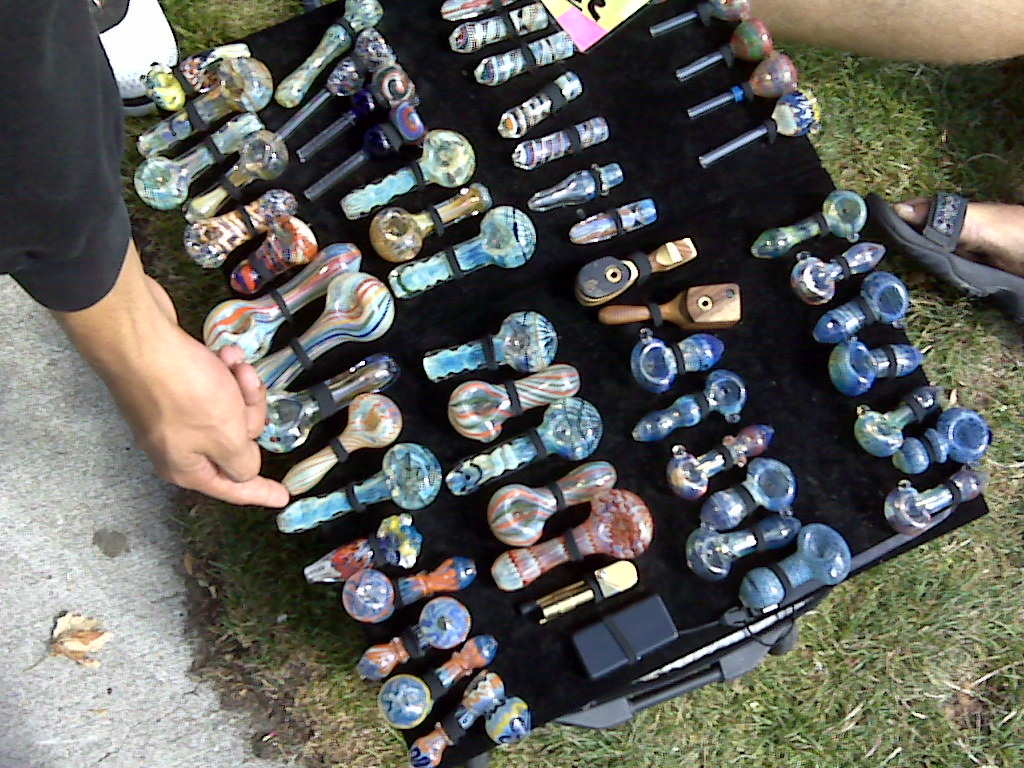The image captures a compelling scene of a meticulously arranged display of approximately 40-50 glass pipes, typically used for smoking marijuana. These pipes, primarily crafted from blown glass and featuring intricate swirling colors, are laid out in four rows on a black background, secured by small elastic bands. Among the predominantly glass pipes are a couple of wooden ones, exuding an old-fashioned charm, and some mouthpieces for bongs. A person in a long-sleeved black shirt is seen pointing to one of the pipes, suggesting a salesperson demonstrating the wares. On the right side of the image, a pair of legs in Teva-like sandals rests on the grass, while in the background on the left, a glimpse of a gray sidewalk with a single leaf can be seen, adding a touch of the outdoors to the setting.